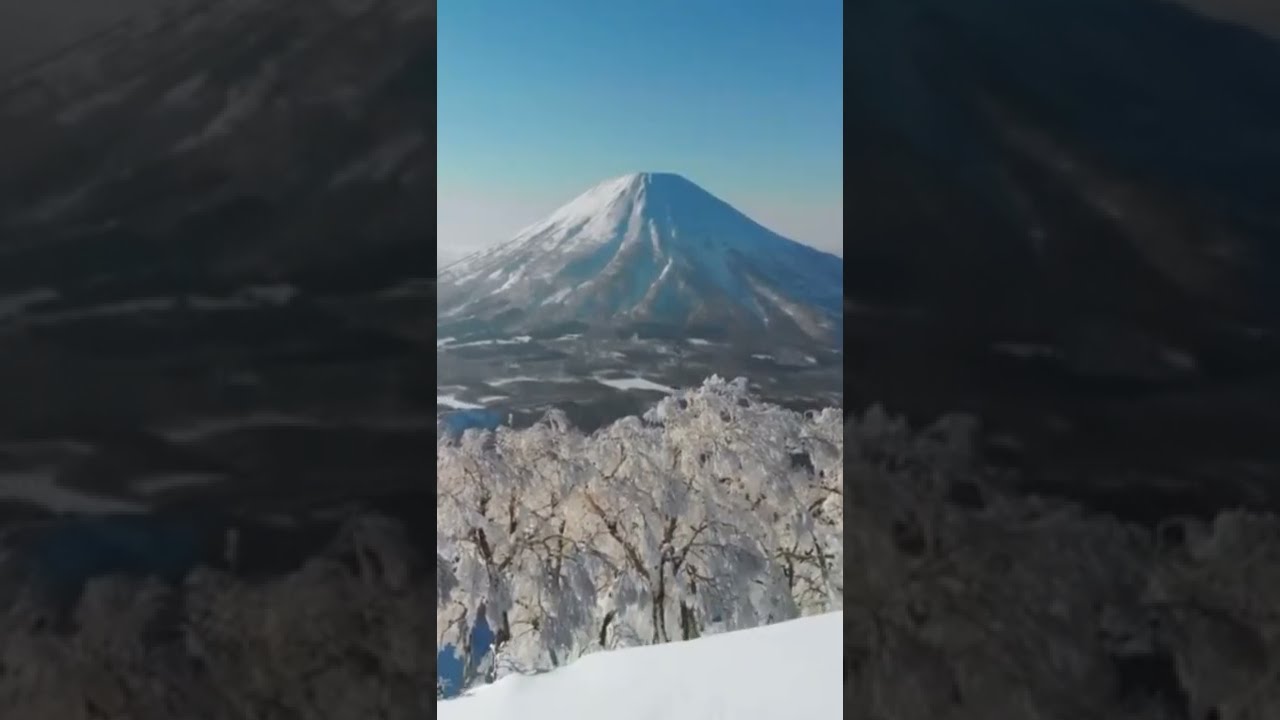In the image, we see a snowy, mountainous landscape captured during the middle of the day. The scene, likely taken from a hilltop, features a serene winter setting devoid of any text. The foreground consists of a layer of snow covering the ground and several small trees or bushes, all heavily blanketed in snow. As we move further up the image, the landscape becomes flat before revealing a large, imposing mountain. The mountain's base and sides exhibit a deep gray hue with sporadic patches of green vegetation, likely trees. However, the mountain's summit is fully enveloped in snow, which cascades down its rounded top and sides in smooth trails. Above the mountain, the clear blue sky is lightly dotted with clouds, adding to the chilly atmosphere of this outdoor scene. The prevalent colors include shades of blue, white, gray, brown, and patches of green, collectively painting a vivid picture of a cold mountainside in winter.